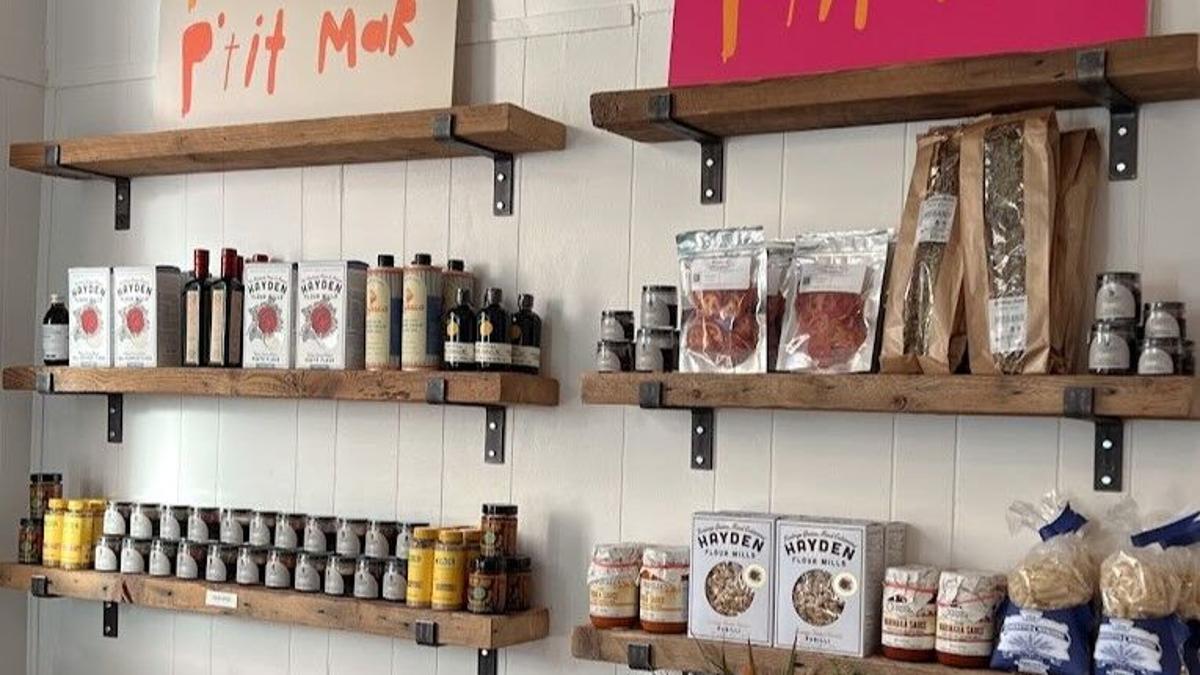The photograph captures a display section featuring a white, vertically paneled wall adorned with six dark brown wooden shelves arranged in two columns of three. Each shelf is supported by black brackets. At the top of the columns, there are signs with orange painted letters, one reading "PITMAR" on a white background and another partially readable sign with similar lettering. The top left shelf houses two white square boxes with identical print, accompanied by two tall bottles with black caps, and two short dark glass bottles featuring white labels at the bottom. On the middle left shelf, more white boxes are flanked by two tall bottles with black caps, and smaller glass jars. The middle right shelf contains various bags of spices. The bottom shelves are populated with multiple jars, including yellow-lidded jars on either side, and additional glass containers. These shelves primarily display an array of packaged food products, including boxes of pasta and jars of sauce, resembling a well-organized pantry or a store display, with the brand name "Hayden" appearing prominently on several packages.